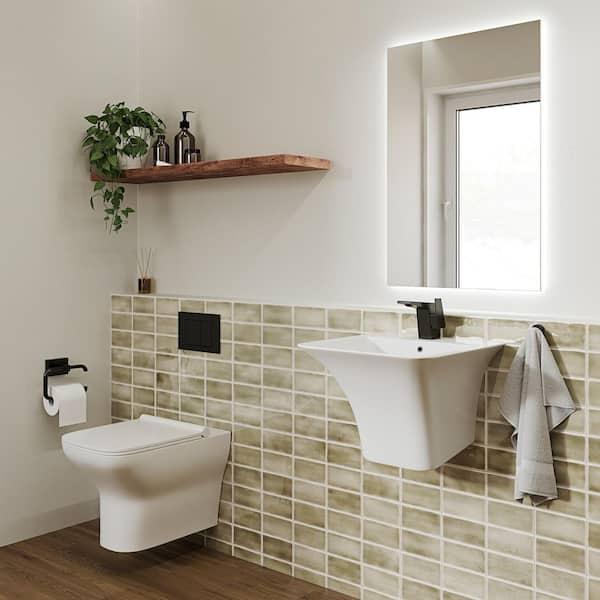This photograph captures a well-lit, modern bathroom with an array of distinct features. The floor is covered in brown wooden planks, extending to meet the tiled walls on the right. The tiles are rectangular, laid in a landscape orientation, and come in shades of gray with white grout. The lower half of the wall showcases these tiles, while the upper half is painted in white. Along the left wall, a white toilet is affixed, complemented by a black square accent and a white toilet paper holder mounted above it. Adjacent to this, on the right wall, there is a white wall-mounted wash basin with a sleek black faucet and a gray towel hanging beside it. Above the sink, a rectangular window emits bright white light, enhancing the bathroom’s airy atmosphere. A wooden shelf positioned over the toilet holds a green plant and three silver bottles, adding a touch of natural decor and modern convenience to the space.